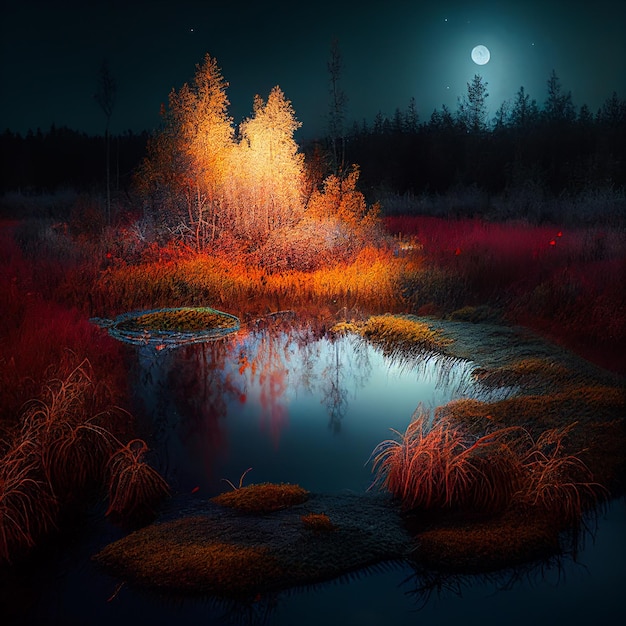In this evocative nighttime scene, we see a serene pond or small puddle under a dark, bluish-gray, silver sky illuminated by a glowing full moon surrounded by a sprinkling of stars. The moonlight casts a gentle glow that permeates the entire setting, highlighting the water's surface and casting intricate reflections of the foliage. Surrounding the pond, closer vegetation is vibrantly lit in hues of red and orange, despite the absence of an apparent light source, while trees and bushes farther away are silhouetted in dark, almost black shades with a touch of gray. The foliage near the water, including small grass pods with bushes on them, radiates with striking red and orange tones, adding depth and color to the tranquil scene. The composition, possibly a painting rendered in acrylic or oil, or even computer-generated, combines detailed, colorful elements with the soft illumination of moonlight, creating a picturesque, almost surreal landscape filled with contrasting shadows and highlighted details.